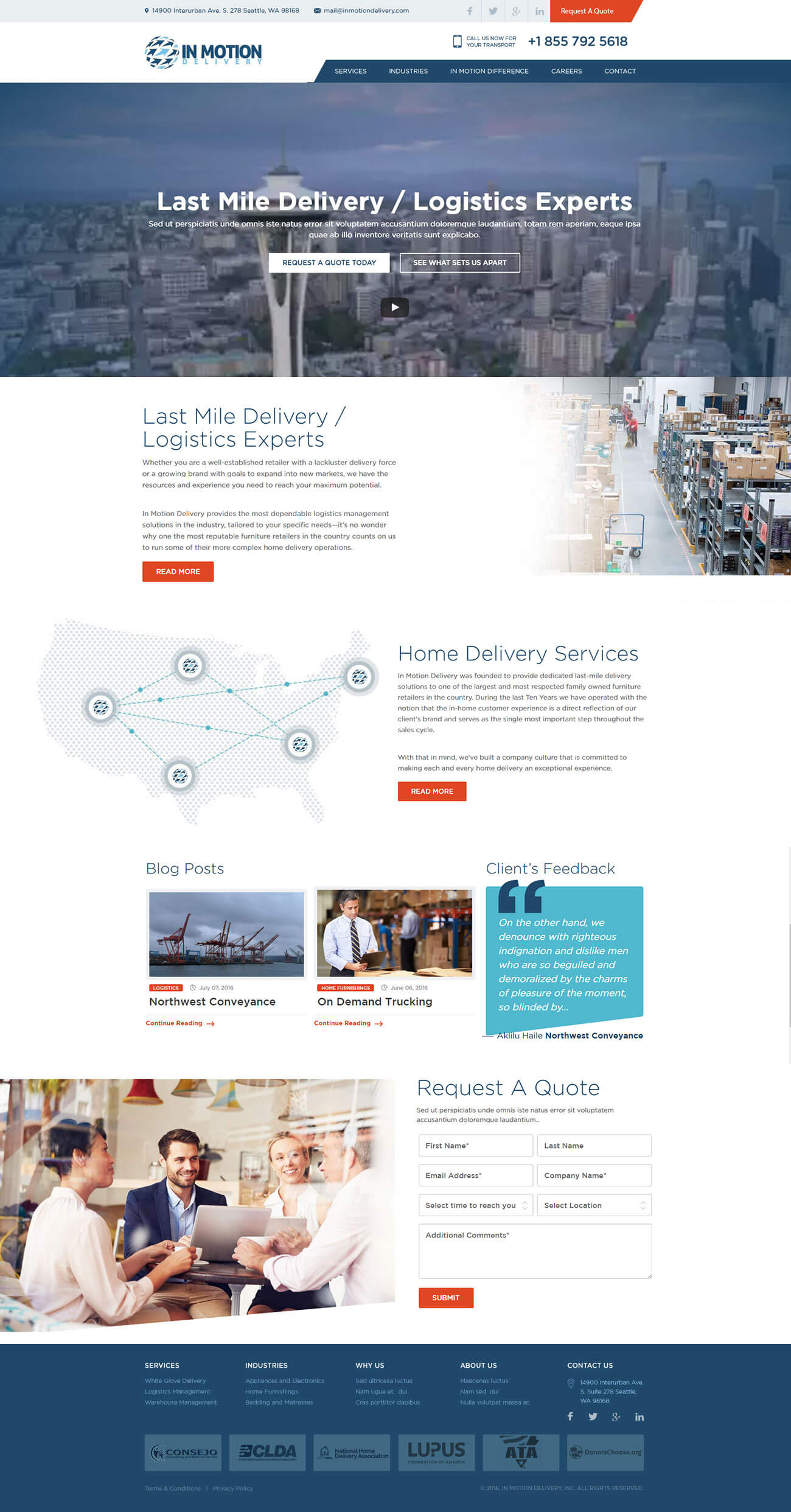The image features a webpage with a predominantly white background, segmented into various sections with distinct colors and elements. At the top, a light blue box transitions into a small red box with very small writing. Below, "In Motion" is prominently displayed alongside a small blue circle surrounded by intricate blue designs. To the right of this, a phone number is listed.

Central to the webpage is a large picture of a dark blue city skyline with tabs at the top. Superimposed on the skyline are the words "Last Mile Delivery / Logistics Experts." Beneath this, there's a white box containing text information about last-mile delivery and logistics services, accompanied by a dark box.

Continuing down, the white background reveals another section reiterating "Last Mile Delivery / Logistics Experts," followed by additional details about these services. Adjacent to this text is a small red button intended for user interaction, and to the right is a small picture depicting a city street.

Further down, a blue-hued map adorned with small circles indicates various locations, highlighted by the label "Home Delivery Services." A red box is present in this section as well. 

There is also a segment titled "Blog Post" featuring two small images, and further down, a section labeled "Clients Restock" within which a small blue box contains more text. Below this, an image captures people sitting around a desk in discussion, and to the right is a "Request a Quote" form with fields for user input and another red button.

At the bottom of the page, a large blue box showcases six different foundation logos, with the only legible one being "Lupus."